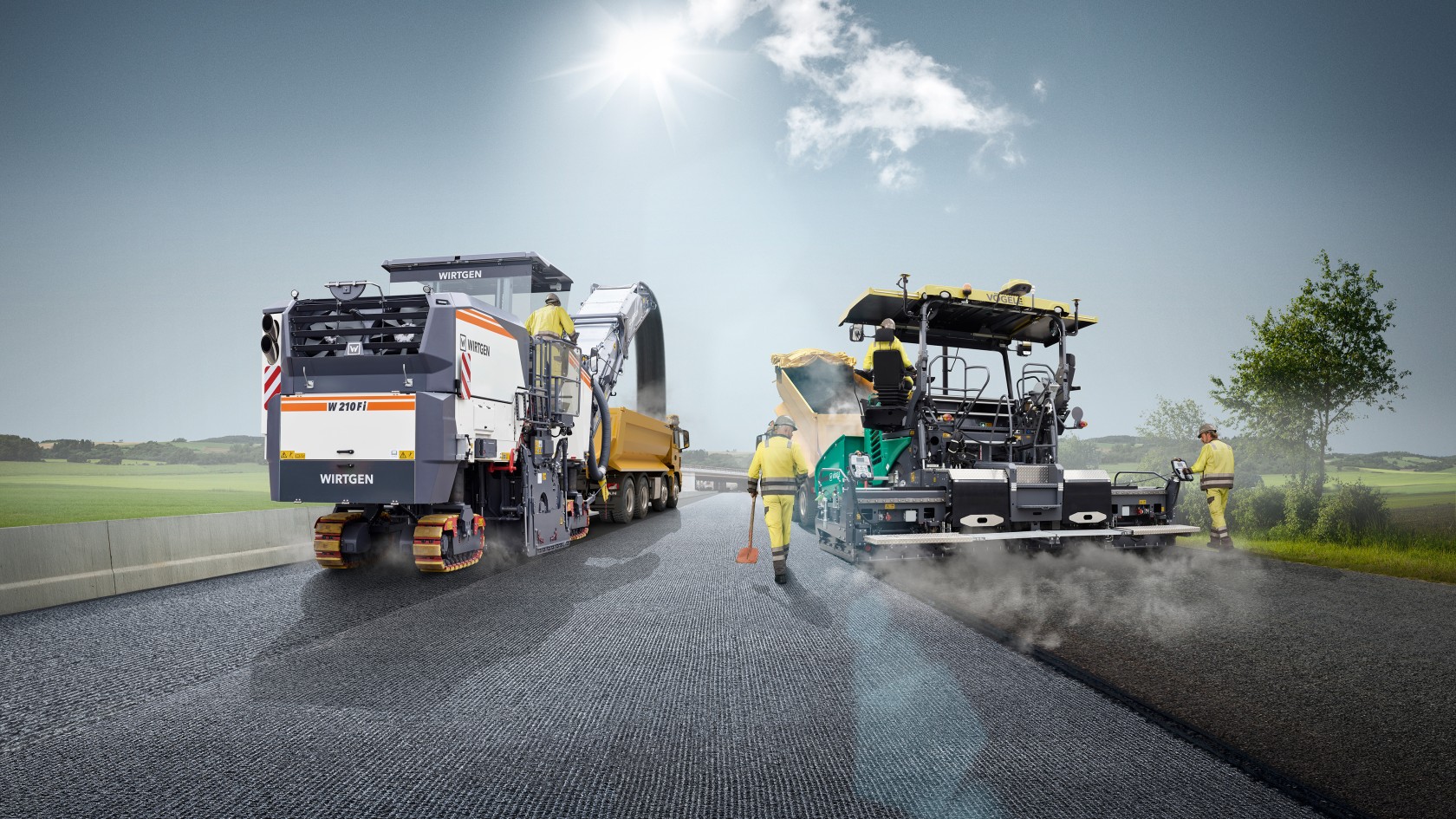The photo appears to be digitally altered due to its near-perfect elements and somewhat unnatural shadows. It captures a scene of road construction, viewed from a low angle looking down a wide, newly paved highway. The pavement is dark charcoal gray with fine lines, creating a very smooth appearance. On the right side, the ground slopes lower, covered with dark gray gravel.

Centered in the image are two large construction machines surrounded by workers in yellow safety equipment and white hard hats. The machine on the right resembles a tractor, emitting steam indicative of hot asphalt, with a man on each side—one holding a tool. Further down, the left side features another large machine, possibly an excavator with orange and white details, feeding stone through a chute into a yellow dump truck. 

Beyond these machines, a yellow dump truck is visible, with what seems to be an operator in yellow safety gear. The landscape is predominantly flat with some distant rolling hills in darker green hues. The sky transitions from a grayish-blue at the top to a lighter color near the horizon, with a bright white sun casting a hazy light over the scene, accompanied by a puffy cloud to its right.